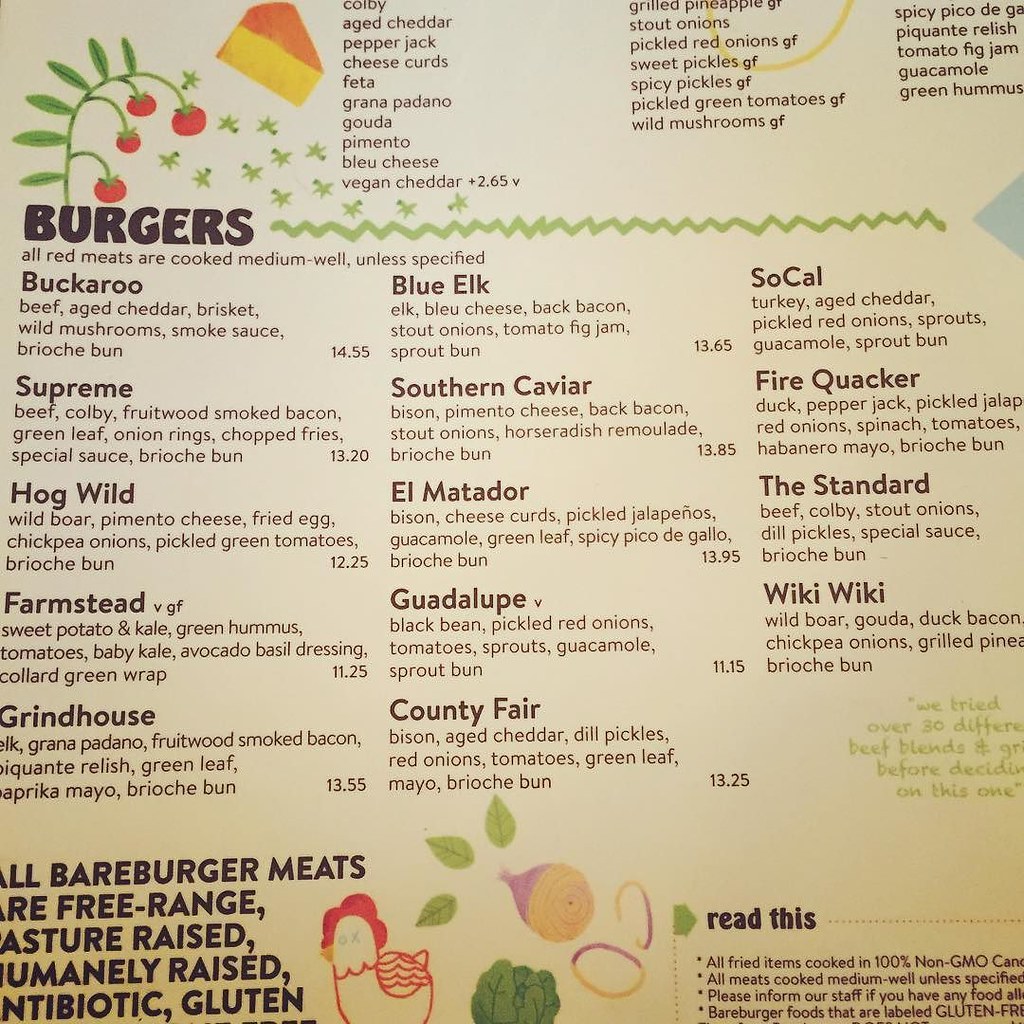The image depicts a section of a specialty burger restaurant menu, prominently featuring a diverse array of burgers. The background of the menu is yellowish, adorned with decorative illustrations of tomatoes or berries, and a green line symbolizing a grassy field. This section focuses on the restaurant's burger offerings, emphasizing the variety of meats and unique ingredients used.

A note specifies that all red meats are cooked to a medium-well doneness unless otherwise requested. The menu showcases around 15 different burgers, including:

- **Buckaroo**
- **Supreme**
- **Hogwild** (wild boar)
- **Farmstead**
- **Grindhouse**
- **Blue Elk** (elk and blue cheese)
- **Southern Caviar** (bison, pimento cheese, back bacon)
- **El Matador** (bison)
- **Guadalupe** (black bean)
- **Fire Quacker** (duck)

The text highlights that all the burger meats are free-range, pasture-raised, humanely raised, antibiotic-free, and gluten-free, emphasizing the restaurant's commitment to quality and ethical sourcing. The price range for these specialty burgers falls between $11 and $15.